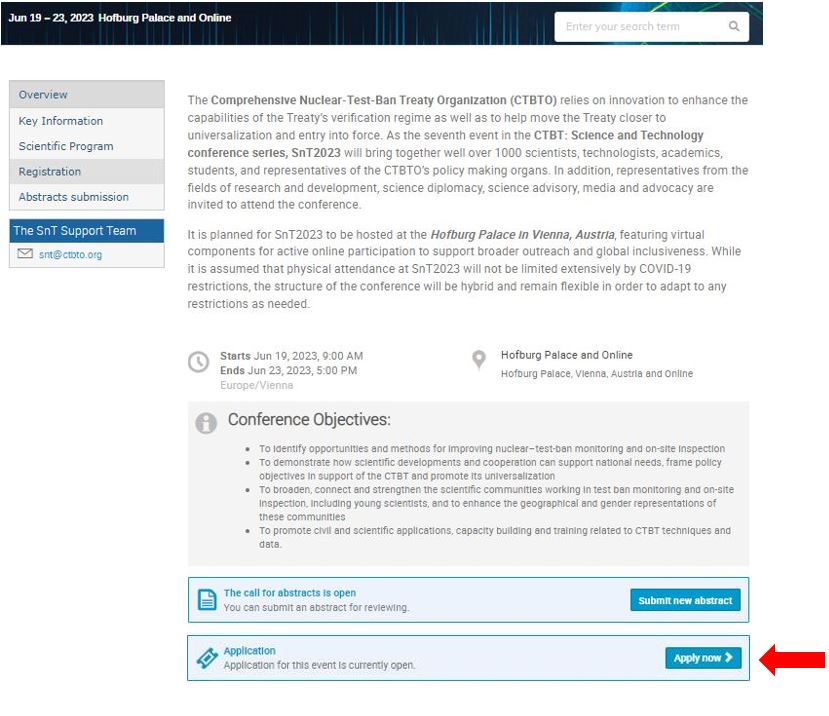The image depicts a detailed webpage design for the Comprehensive Nuclear Test Ban Treaty Organization (CTBTO) Science and Technology Conference (SNT) 2023. 

**Top Border:**
- The very top border of the page features a dark color with patches of black interspersed with green or bluish vertical lines.
- In the upper left corner, the date "June 19 to 23, 2023" is displayed in white, along with the venue details: "Hofburg Palace and online."
- On the far right, there is a white search bar with light gray text that reads "Enter your search here" accompanied by a magnifying glass icon.

**Left-Hand Side Menu:**
- Below the top border, the left-hand side of the webpage contains a menu:
  - The first item is a gray bar labeled "Overview" in blue text.
  - The second item is a white bar labeled "Key Information."
  - The third item is a white bar labeled "Scientific Program."
  - The fourth item is a gray bar labeled "Registration."
  - The fifth item is a white bar labeled "Abstract Submissions."
  - Below these items, there is a blue label with white text that reads "The SNT Support Team."
  - Underneath this, a white section features an envelope icon along with a partially legible email address ending in ".org" for the SNT support team.

**Main Content Area:**
- To the right of the menu, the background is white with grayish-black text containing detailed information about the conference.
- The text describes the CTBTO's reliance on innovation to enhance the treaty verification regime and efforts to move the treaty closer to universalization and entry into force.
- The conference, labeled as SNT 2023, aims to gather over 1,000 participants including scientists, technologists, academics, students, and CTBTO policy representatives.
- Additional invitees include individuals from research & development, science diplomacy, science advisory, and media advocacy.

**Event Schedule and Location:**
- Below the main text, a clock icon indicates the schedule: June 19, 2023, at 9 a.m. to June 23, 2023, at 5 p.m. (Europe-Vienna time).
- A location icon shows the physical and virtual venues: Hofburg Palace in Vienna, Austria, and online.

**Conference Objectives:**
- Following the event details, a grayish box with a circle containing an "i" icon lists the conference objectives, including:
  1. Identifying opportunities and methods for improving nuclear test monitoring and on-site inspection.
  2. Demonstrating how scientific development and cooperation can support national needs, policy objectives, and CTBT promotion.
  3. Broadening and strengthening the scientific communities engaged in test ban monitoring and on-site inspection, focusing on young scientists.
  4. Enhancing geographical and gender representation within these communities to promote civil scientific applications, capacity building, and training related to CTBT techniques and data.

**Additional Conference Information:**
- Below the objectives, a blue section features a document icon with the message "The call for abstract is open. You can submit an abstract for review."
  - Adjacent to this message, a blue button with white text says "Submit New Abstract."
- Another blue box further down contains a ticket icon that states "Application for this event is currently open."
  - To the right of this message, a blue button with white text reads "Apply Now," emphasized by a red arrow pointing to it.